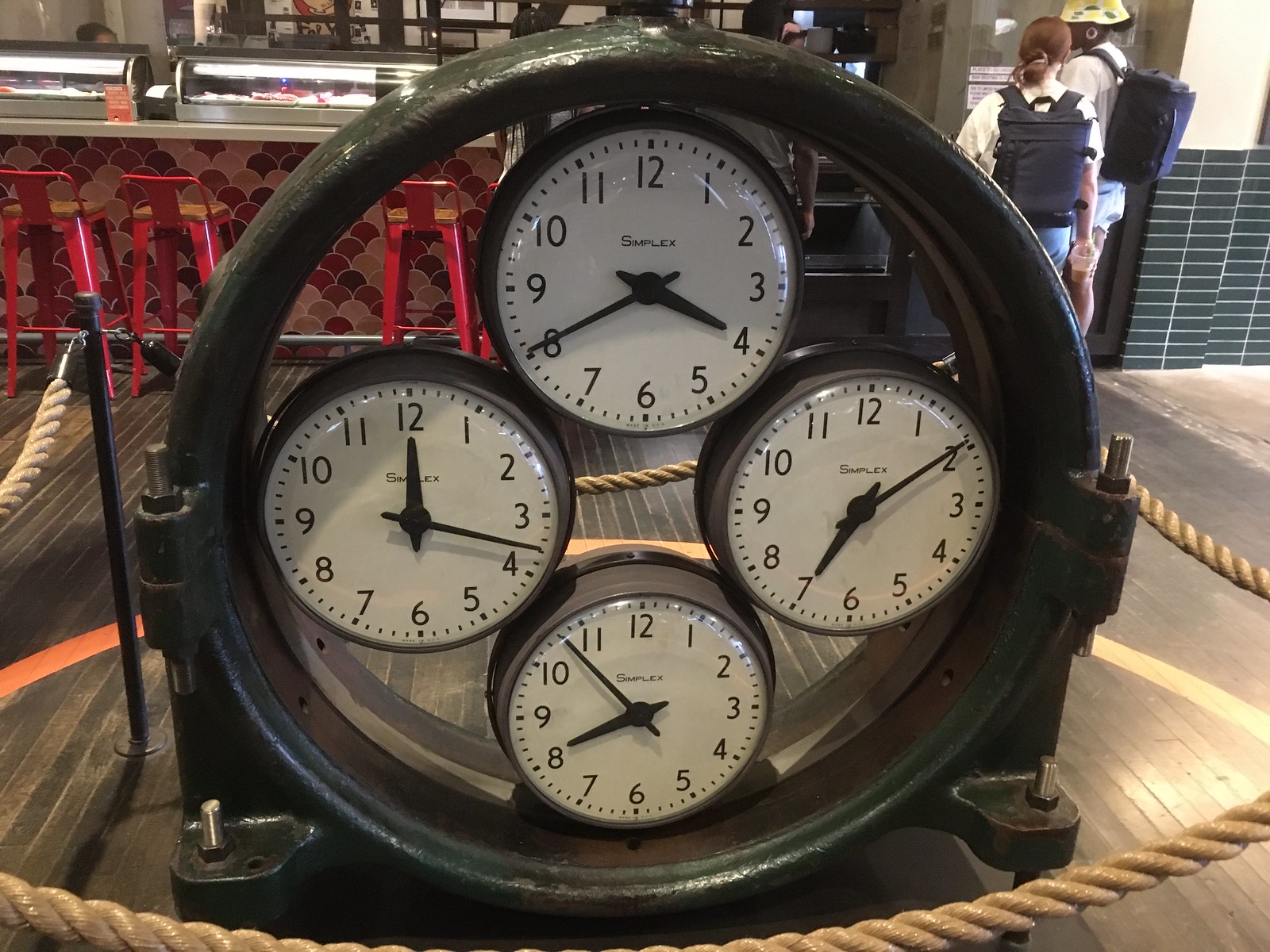This image captures a vintage clock display featuring four small, circular timepieces arranged in a circular frame. Each clock displays a different time, yet they all share the central text "Simplex" and utilize a standard 1 to 12 numbering system. The background reveals a food service area, characterized by bar chairs and illuminated food containers. A few people are visible towards the right, carrying large backpacks, indicating this might be a bustling tourist location.